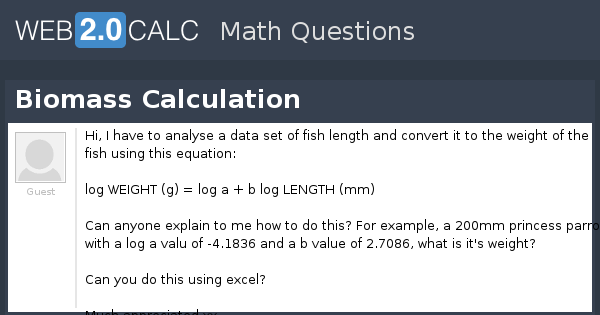This image depicts a partial screenshot of a website, prominently showing a section dedicated to solving math problems. At the top of the image, within a blue box, the term "2.0" is displayed in bold white font. Adjacent to this, the site is titled "C-A-L-C" (Calc). Centered below this header, in a gray banner, the phrase "Math Questions" is visible.

Further down, there is a horizontally spread black rectangular area. Beneath this, the text "Biomass Calculation" is clearly shown. 

The main section of the page consists of a white background with a format featuring a user input interface. On the left side, there is a placeholder labeled "Guess," accompanied by an empty profile picture frame. A vertical line divides this segment from the textual content on the right.

The text on the right reads: "Hi, I have to analyze a dataset of fish lengths and convert it to the weight of the fish using this equation: log(weight in g) = log(a) + b*log(length in mm)." Following this introduction, the user inquires, "Can anyone explain to me how to do this? For example, a 200 mm [fish] with log..." and proceeds to detail the equation further before asking, "Can you do this using Excel?"

This comprehensive caption captures the essence and details of the website's interface and the user's query.